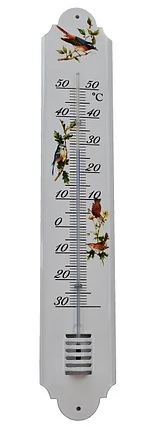In this image, the background is entirely white, creating a seamless and borderless effect that extends across the screen. At the center stands a vertically oriented thermometer, which appears to be part of a product display, given that it is not mounted to any visible background element.

The thermometer itself is off-white in color and features a distinctive shape. It is primarily rectangular but tapers slightly towards both ends. At the top and bottom, the shape transitions into a small inward-arching curve, culminating in an oval "bubble." These bubbles, one at each end, both contain a small hole likely intended for hanging the thermometer.

The face of the thermometer is adorned with numerical markings and dashes. The Fahrenheit scale is situated on the left-hand side, ranging from -30 up to 50 degrees. The Celsius scale occupies the right-hand side, displaying numbers up to 50 degrees, but curiously omits negative values.

Adding a touch of charm, there are four decorative birds positioned along the thermometer's length, providing a whimsical and visually appealing element to the otherwise functional design.